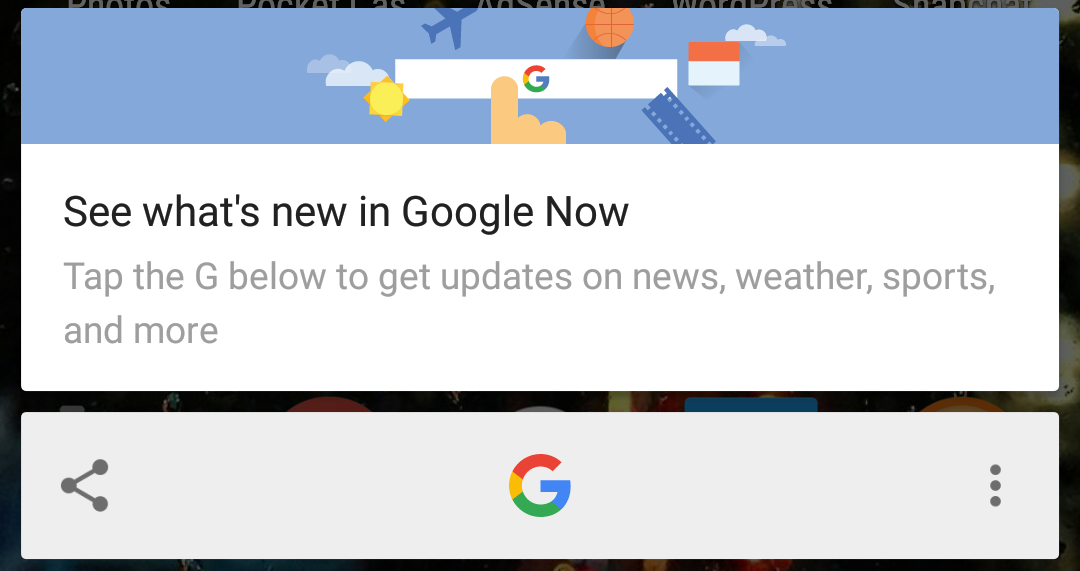The image depicts a pop-up notification appearing on someone's screen. The pop-up prominently features a light blue banner at the top, showcasing a central illustration of Google's "G" logo. Surrounding this logo are whimsical, hand-drawn icons including an airplane, a basketball, a film strip, a finger, a sun, and a couple of clouds, all contributing to a playful and engaging presentation. 

The focal text, "See what's new in Google now," is rendered in bold black font, commanding attention. Below this, finer print reads, "Tap the G below to get updates on news, weather, sports, and more," guiding the user on further action. At the bottom of the pop-up, within a larger box, sits the iconic, multicolored Google "G" (red, yellow, green, and blue), indicating an actionable button likely leading to a search bar or Google’s service updates.

The backdrop behind this pop-up is indiscernible, appearing to be a photograph with darker hues and minimal prominent whites, which further directs focus onto the vibrant and inviting pop-up interface.